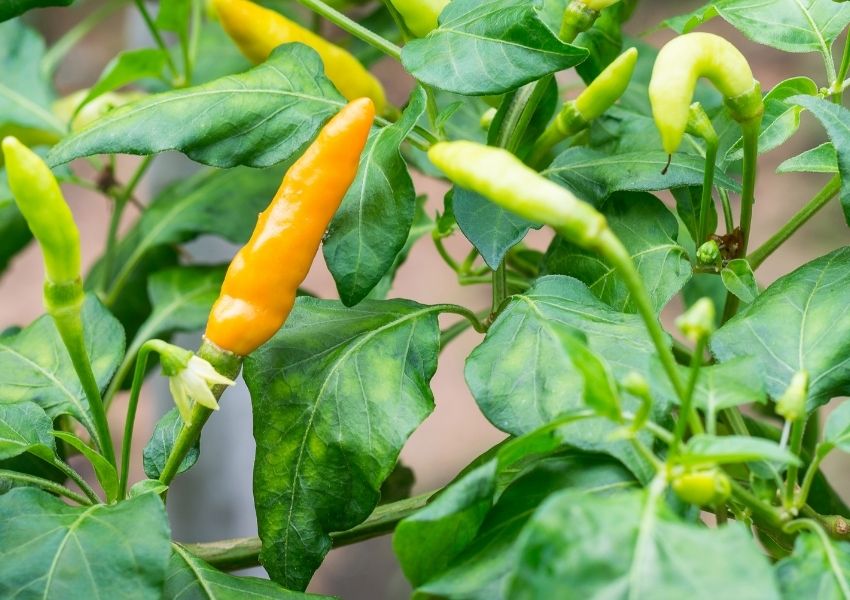This detailed photograph captures a close-up view of a pepper plant set against a blurred, indistinct beige background. The canvas of the image is filled with foliage, showcasing a mix of dark green and lime green leaves. Dominating the foreground are several pepper pods in various stages of ripeness. The most prominent is a deep orange pod, positioned at a steep angle from the bottom left upward, highlighted with white on its upper surface and shaded underneath. To its left is a smaller, green pod, and to the right, there are two more green pods, one angled at 45 degrees in the center of the frame and another drooping slightly in the top right corner, with a small black tip resembling a stem. The background features a hint of darker objects shrouded in a smoky gray haze, ensuring the bright and colorful pods, especially the striking orange one, remain the focal point of this vibrant garden scene.